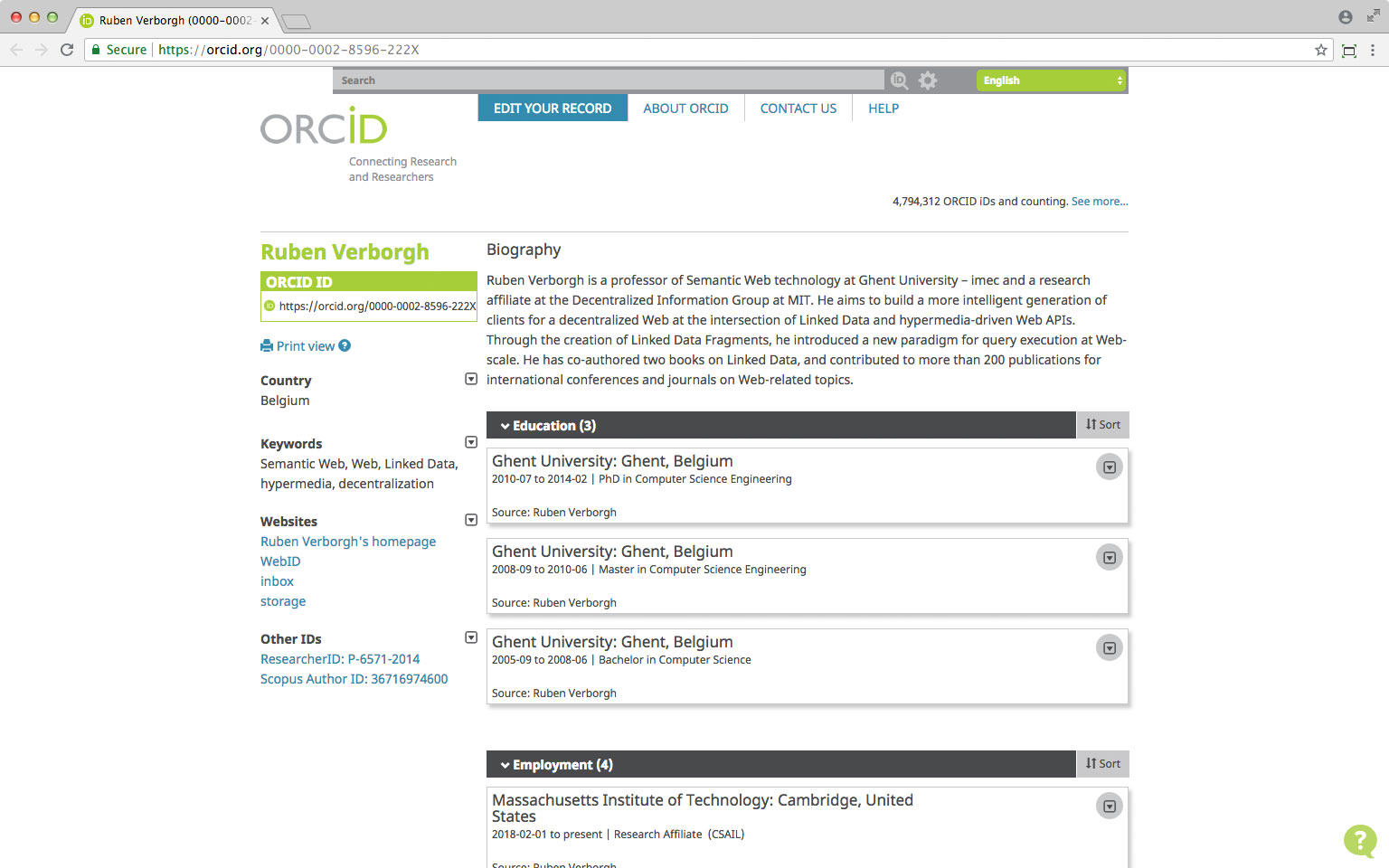This is a screenshot of the ORCID.org website displaying the profile of Ruben Verborgh. As the text is small and somewhat difficult to read, the following details can be discerned:

1. **Header**: The website's header prominently displays "ORCID.org."
2. **Profile Name**: Featured at the top is the name Ruben Verborgh, identified as a Professor of Semantic Web Technology at Ghent University.
3. **Institution**: Ghent University, located in Belgium, is highlighted with details indicating his affiliation and employment history.
4. **Employment**: Includes a notable position at the Massachusetts Institute of Technology (MIT) in Cambridge, United States.
5. **Keywords**: Key topics associated with Ruben Verborgh include "web," "web link data," "hypermedia," among others.
6. **Additional Sections**: The left side of the profile lists various sub-sections such as:
   - **Websites**: Four different personal or professional websites are linked.
   - **IDs**: Includes ORCID ID, inbox, storage, other IDs, Researcher ID, and Scopus Author ID.
7. **Navigation Options**: There are several navigational links available for users, such as:
   - **Edit Record**
   - **About ORCID**
   - **Contact**
   - **Help**: Suggested for additional support or understanding the platform.
   
Overall, the image captures a comprehensive yet intricate layout of an academic profile on ORCID.org, emphasizing affiliations, key thematic interests, and various professional identifiers.